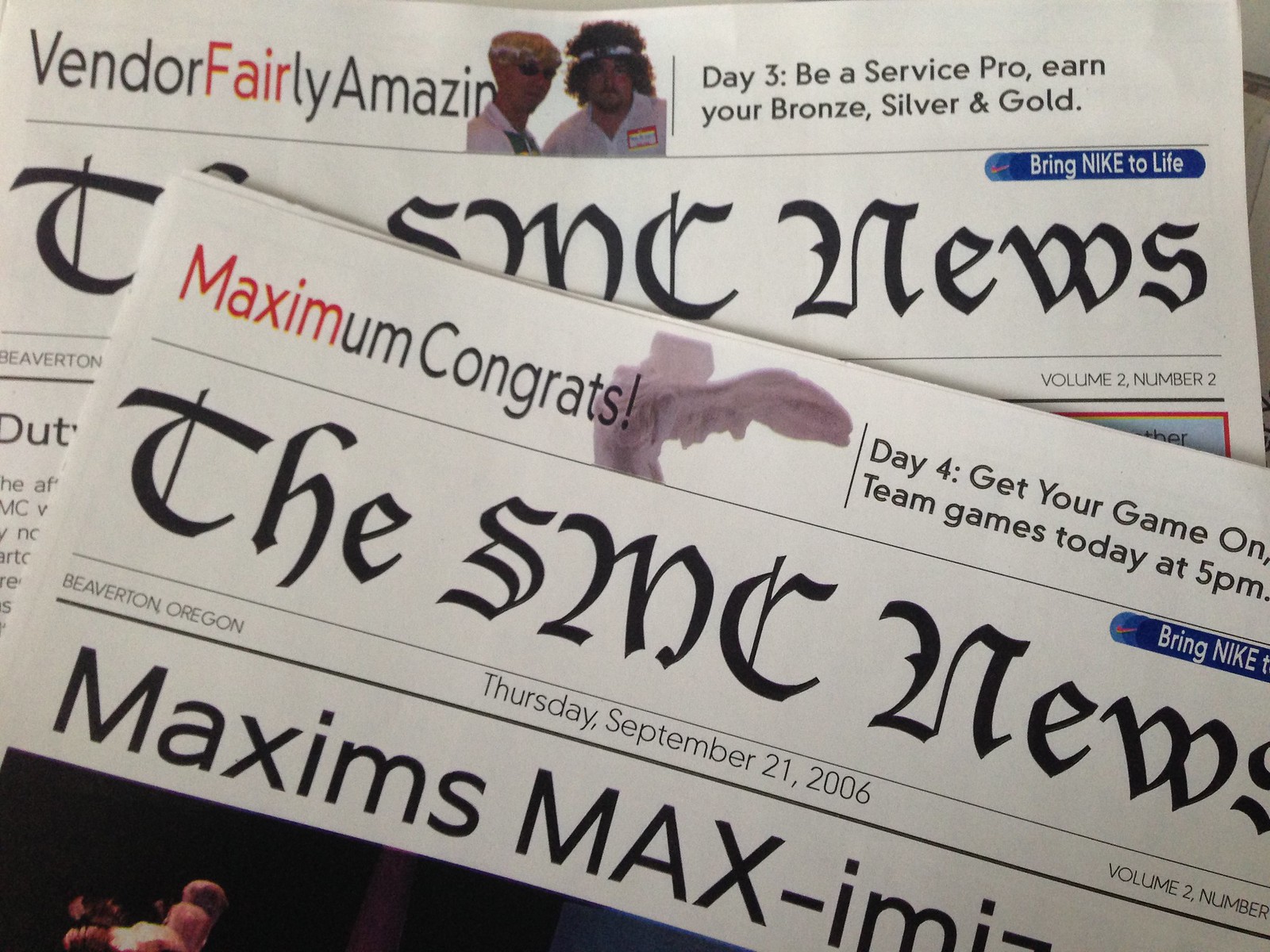The image shows two overlapping newspapers from SMC News. The newspaper on the top is titled "Maximum Congrats," dated Thursday, September 21, 2006. This edition features headlines such as "Day 4 - Get Your Game On" and "Team Games Today at 5 p.m." The publication emphasizes the title "Maximize" and hails from Beaverton, Oregon. Beneath it, the second newspaper is partially visible with the title "Vendor Fairly Amazing," highlighting "Day 3 - Be A Service Pro, Earn Your Bronze, Silver, and Gold." Both newspapers appear layered, concealing some of the information, but still providing a glimpse of their vibrant headlines and shared theme of motivational and community-focused events.